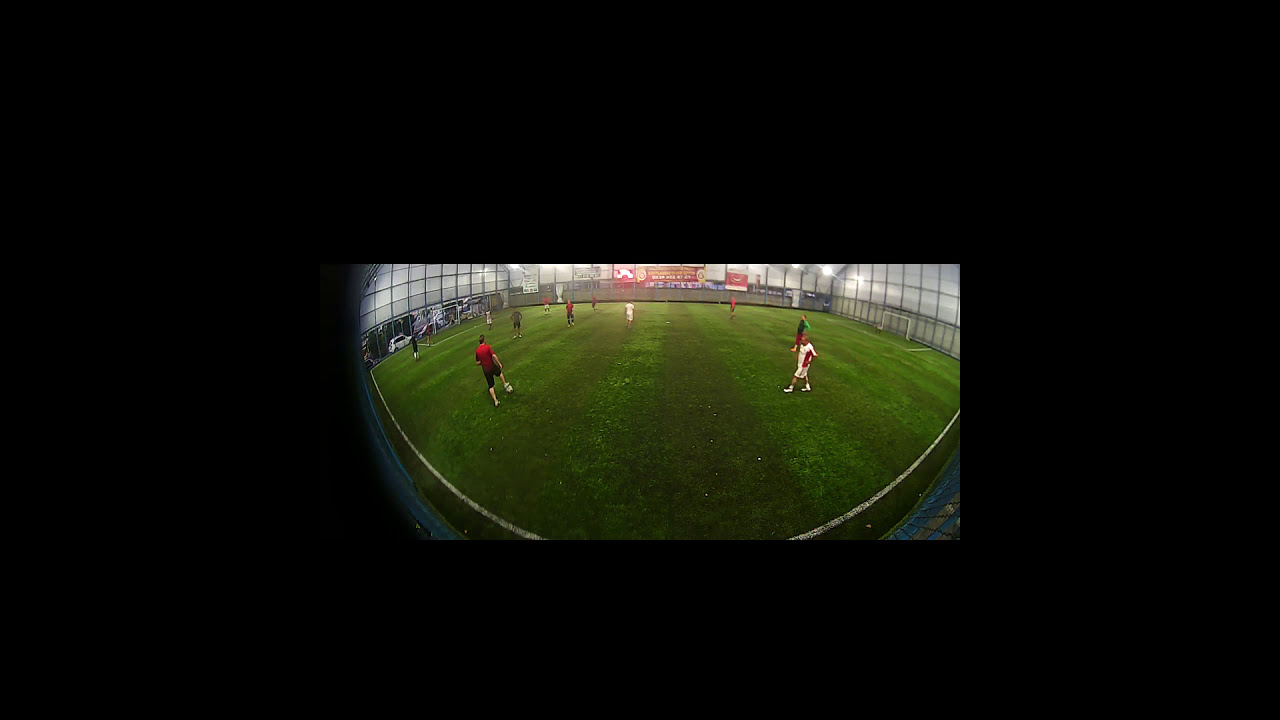This photograph captures an indoor soccer match framed within a large black border that occupies most of the image. The smaller, inner frame - about a third of the image's height and half its width - is centered and showcases a bright green field with striped turf, indicative of either natural grass or artificial turf. The image is slightly distorted by a convex lens, creating a curvature from left to right.

In the inner frame, two teams can be seen: one in red jerseys and the other in white. On the left side of the field stands a player in a red jersey, while a player in a white jersey is positioned to the right. Additionally, a person wearing a green shirt, likely a referee or goalie, is also visible. The distant mid-ground reveals more players dressed in the respective team colors, along with two soccer goals placed on opposite ends of the field. 

The venue appears to have frosted glass windows that let in diffused light while obscuring the outside view. Signage adorns the far wall, and a scoreboard is lit up, adding to the indoor arena's ambiance. The panoramic distortion, wide-angle view, and detailed surroundings highlight the dynamic nature of the indoor soccer match.